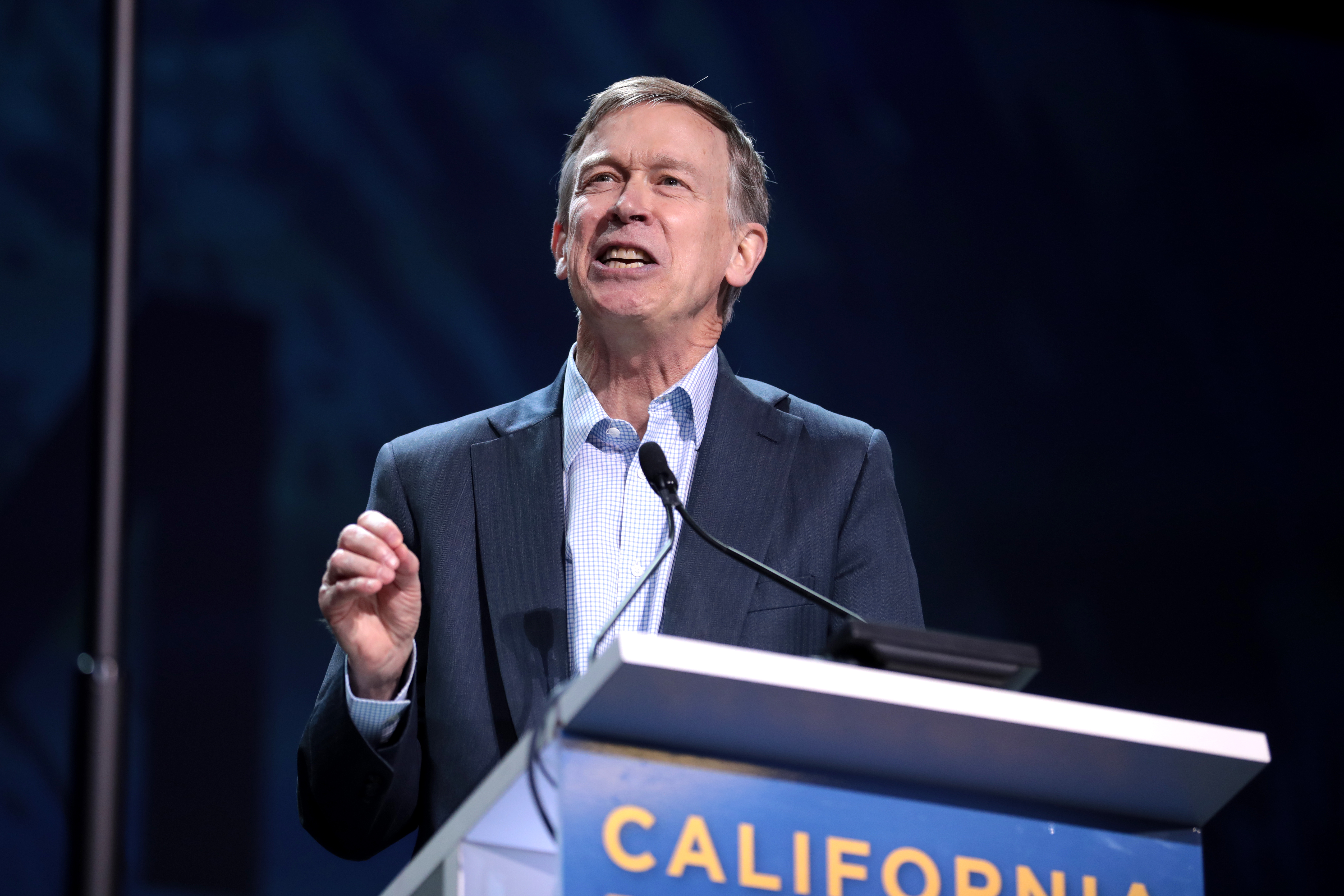The photograph captures a distinguished-looking man, possibly a politician or commentator, standing behind a prominently placed white wood podium with a blue placard bearing the partially visible yellow text "California." Multiple wires run from behind the placard to two microphones positioned toward the man's face. He is mid-speech, appearing passionate and emphasizing a point with his raised right hand, where his index finger, middle finger, and thumb touch as part of a gesture; his left hand is out of view below the podium.

The man, likely in his mid to late 50s or early 60s, is well-groomed with short gray hair. He wears a light blue and white checkered button-up shirt with an open collar, topped by a darker blue sports jacket. His gaze is directed slightly upward and to the left. Behind him, a solid dark blue backdrop completes the scene, along with a pole positioned to the right of him (viewer's left). Despite the blurred background, the focus is clearly on his impassioned expression and authoritative presence at the podium.